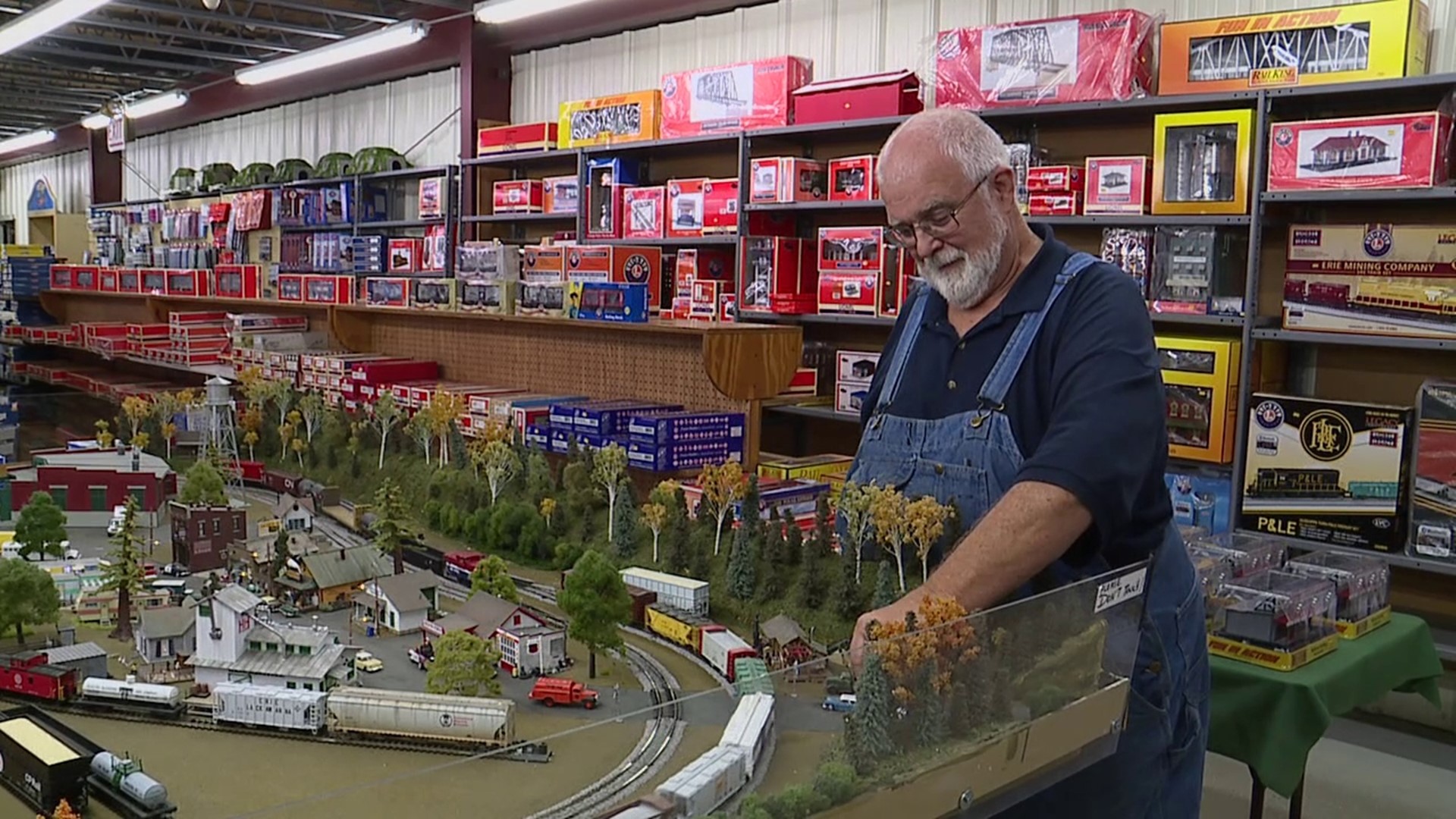The image depicts an older gentleman in a hobby shop or model train store, engrossed in adjusting a large, intricately detailed model train set. He is wearing light blue denim overalls over a navy short-sleeve collared shirt, complemented by black-rimmed glasses. His appearance is characterized by short white hair, a white beard, and a balding forehead. The model train set he is working on is housed within a large enclosure featuring model trains, cars, trees, houses, and other miniature elements, all meticulously arranged to create a lifelike village scene. His hand is partially hidden by the fake evergreens as he touches or adjusts one of the train cars. Surrounding him and behind the green table in the background are numerous shelves stocked with box sets of model trains and various accessories, enhancing the impression of a well-stocked hobbyist's paradise. The space is well-lit with ceiling lights, illuminating both the man and the extensive array of train goods.